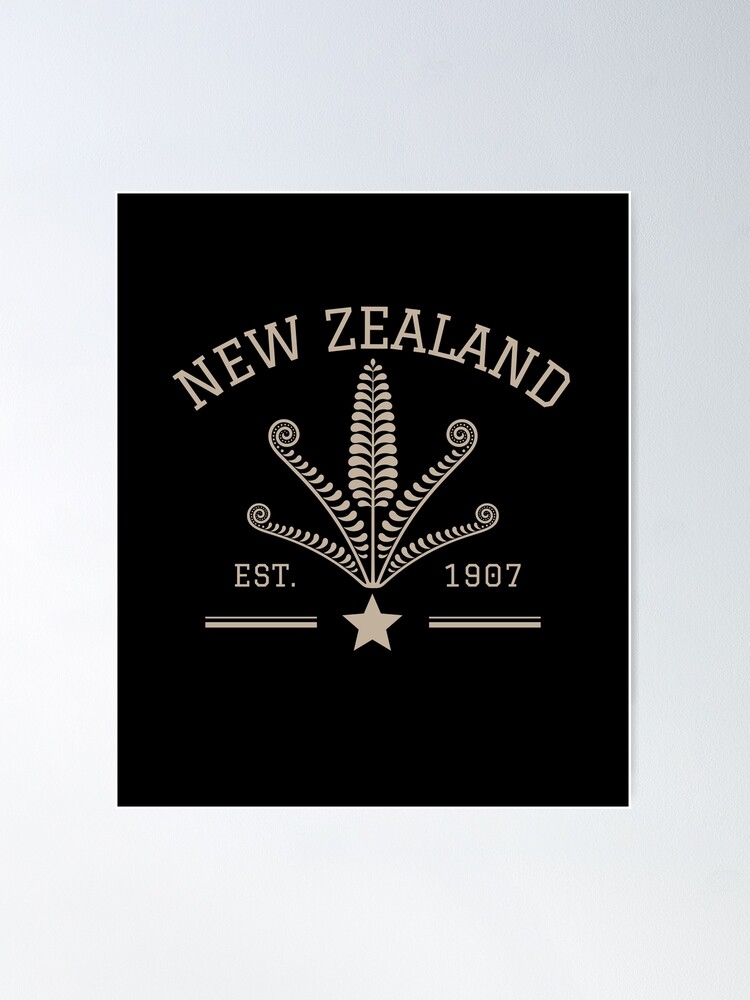The image features a black background adorned with goldish-yellow lettering and designs. At the top, the text "New Zealand" is prominently displayed in large, curving letters that taper downwards towards the edges. Central to the design is an ornate, plant-like emblem resembling a stem of wheat or a floral stalk, complete with multiple dense leaves extending symmetrically on both sides. To the left of this emblem, near the base, the text reads "EST." while to the right, "1907" is inscribed, both accompanied by horizontal lines beneath them. At the very bottom of the image, a lone star is positioned centrally, also flanked by horizontal lines. The poster stands out against a grayish border that frames the entire scene.